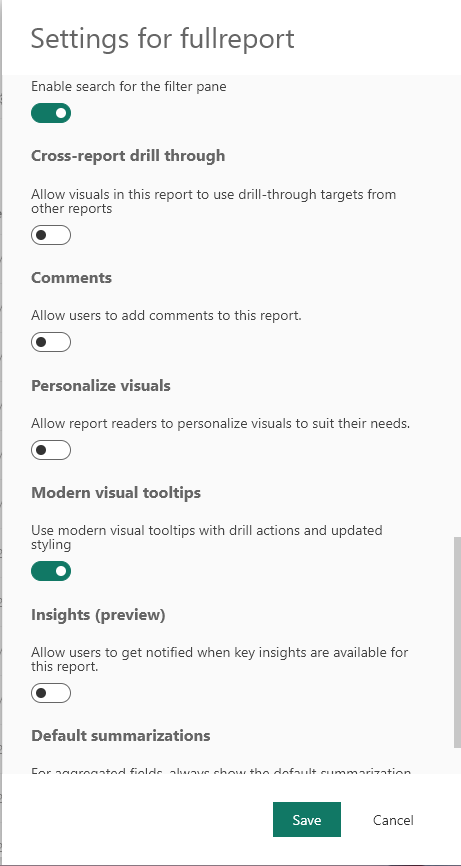In this image, the background is a light purple color. At the top, there is a white box containing the text "Settings for Full Report." Below this, the interface lists various settings each paired with a toggle switch. 

The first setting, labeled in purple, is "Enable search for the filter pane," accompanied by a green toggle switch. Following this is "Cross Report Drill Through," which states, "Allow visuals in this report to use Drill Through targets from other reports." This setting also features a toggle switch. 

Next, the "Comments" section allows users to add comments to the report and includes a toggle switch. Then there is "Personalized Visuals," which permits report readers to personalize visuals according to their needs, again accompanied by a toggle switch. 

The "Modern Visual Tooltips" section describes using updated styling and drill actions for tooltips and also comes with a green toggle switch. 

Below this, the "Insights Preview" setting allows users to get notifications when key insights are available for the report, complete with a toggle switch. 

Lastly, the "Default Summarizations" setting is shown, and at the bottom, there is a white block containing two buttons: a green "Save" button and a white "Cancel" button.